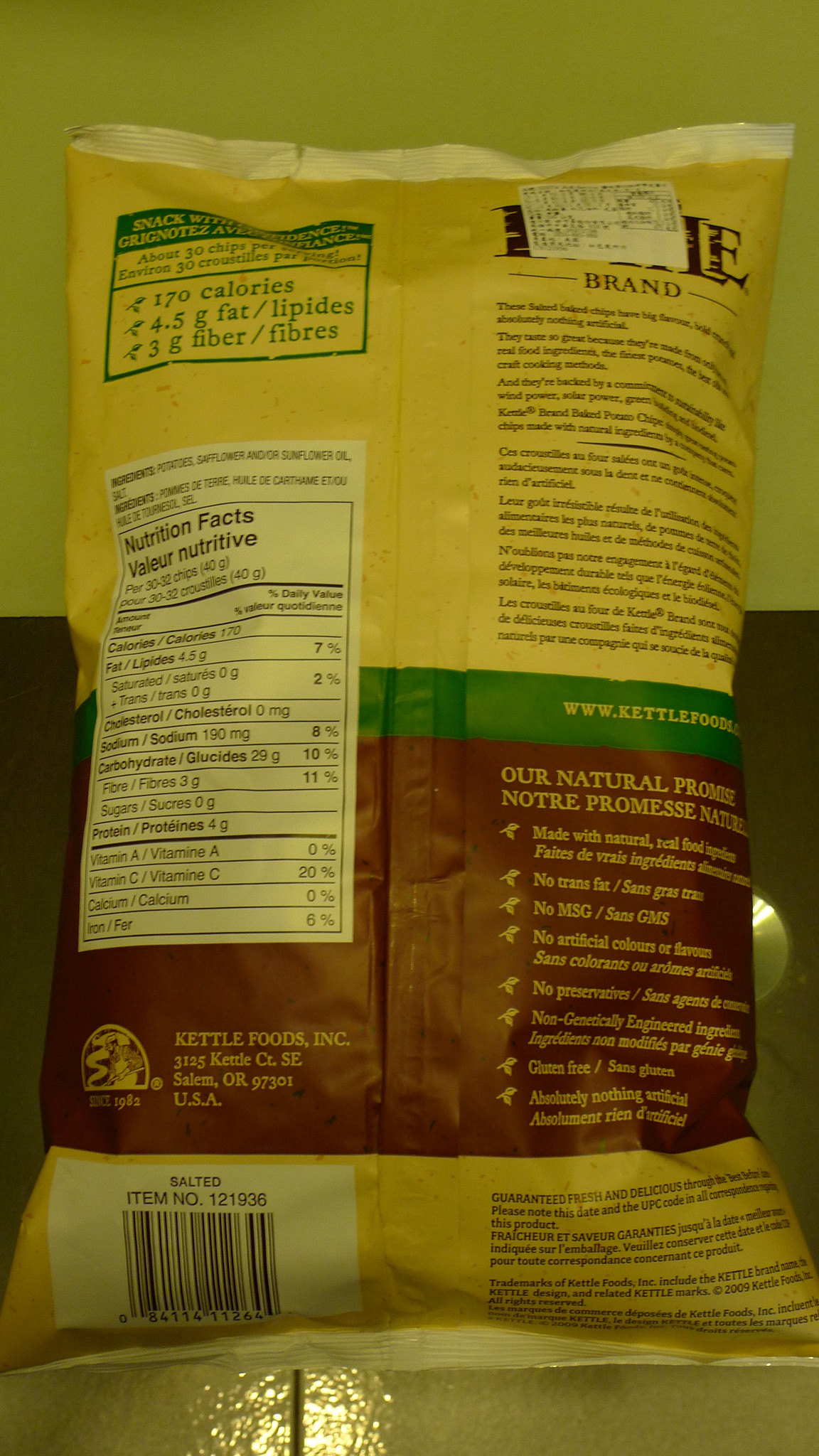This close-up photograph features the back of a bag of Kettle brand chips, produced by Kettle Foods Incorporated. The bag has a yellowish tint, possibly due to lighting or a filter. The bag's design includes a yellow top and bottom, with a green stripe through the middle and a burgundy-brown section below it. The back of the bag is visible, partially obscured by a sticker covering the brand name. The text on the bag details the company's natural promises and attributes, with nutritional information located in the middle-left section. The calorie content is listed in the upper left corner, while the brand's description appears in the upper right. The barcode, set against a white background, is in the lower right corner. The bag is positioned on a shiny beige countertop, with a yellow wall above and a brown section below in the background.